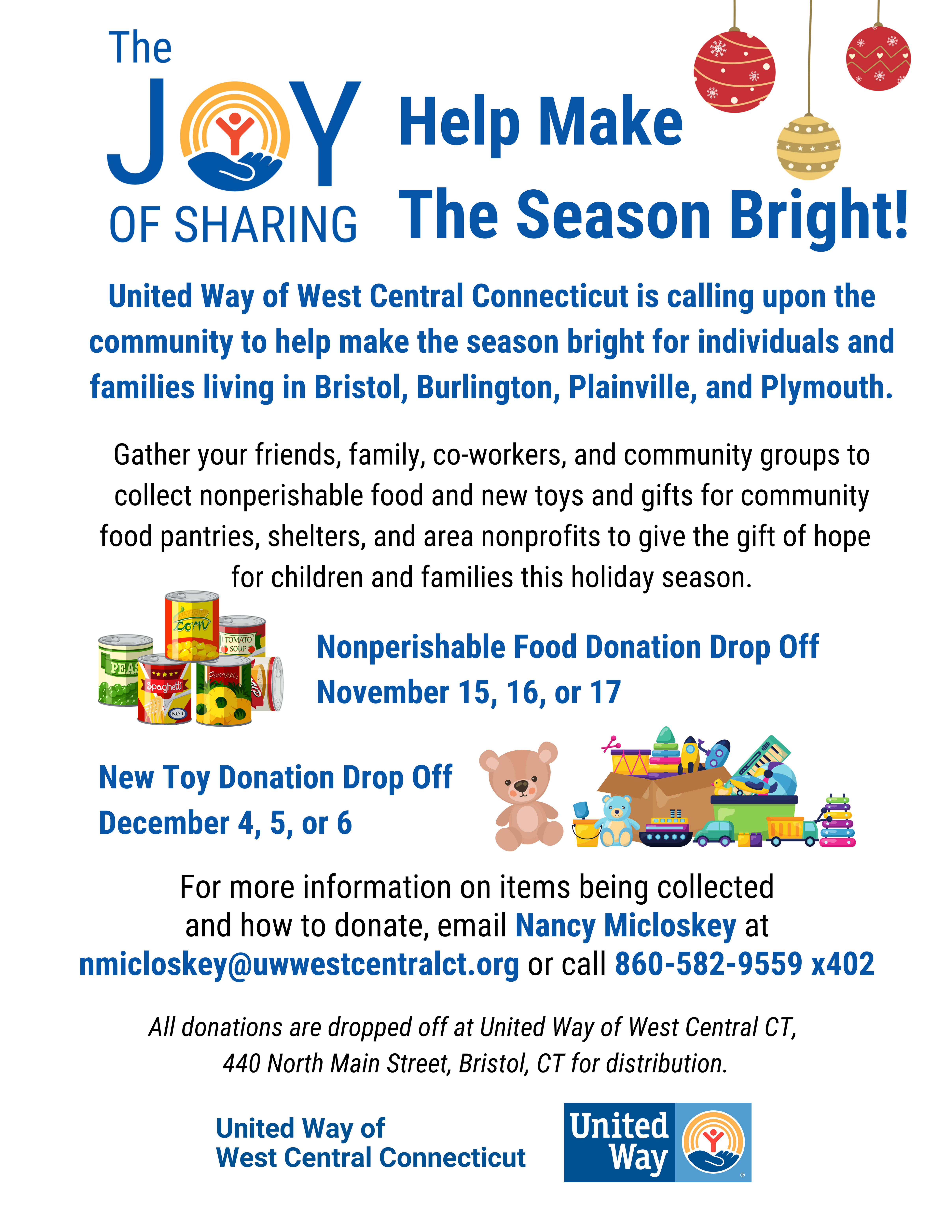This image is a holiday-themed advertisement flyer for the United Way of West Central Connecticut, aiming to bring joy and hope to individuals and families in the Bristol, Burlington, Plainville, and Plymouth areas. Titled "The Joy of Sharing: Help Make the Season Bright," it calls on the community to come together—friends, family, co-workers, and community groups—to collect non-perishable food and new toys or gifts for local food pantries, shelters, and area non-profits. Key details include the following:

- Non-perishable food donations can be dropped off on November 15th, 16th, or 17th.
- New toy donations can be dropped off on December 4th, 5th, or 6th.
- For more information on the items being collected or how to donate, individuals can contact Nancy McCloskey via email at nmccloskey@uwwestcentralct.org or by phone at 860-582-9559, extension 402.

The flyer is visually striking, set against a white background with holiday-themed elements such as Christmas ornament balls, images of canned food, and various toys including a teddy bear. Key information is highlighted in blue text, with additional details in black. The bottom of the flyer features the United Way logo, reinforcing the organization's presence and mission.